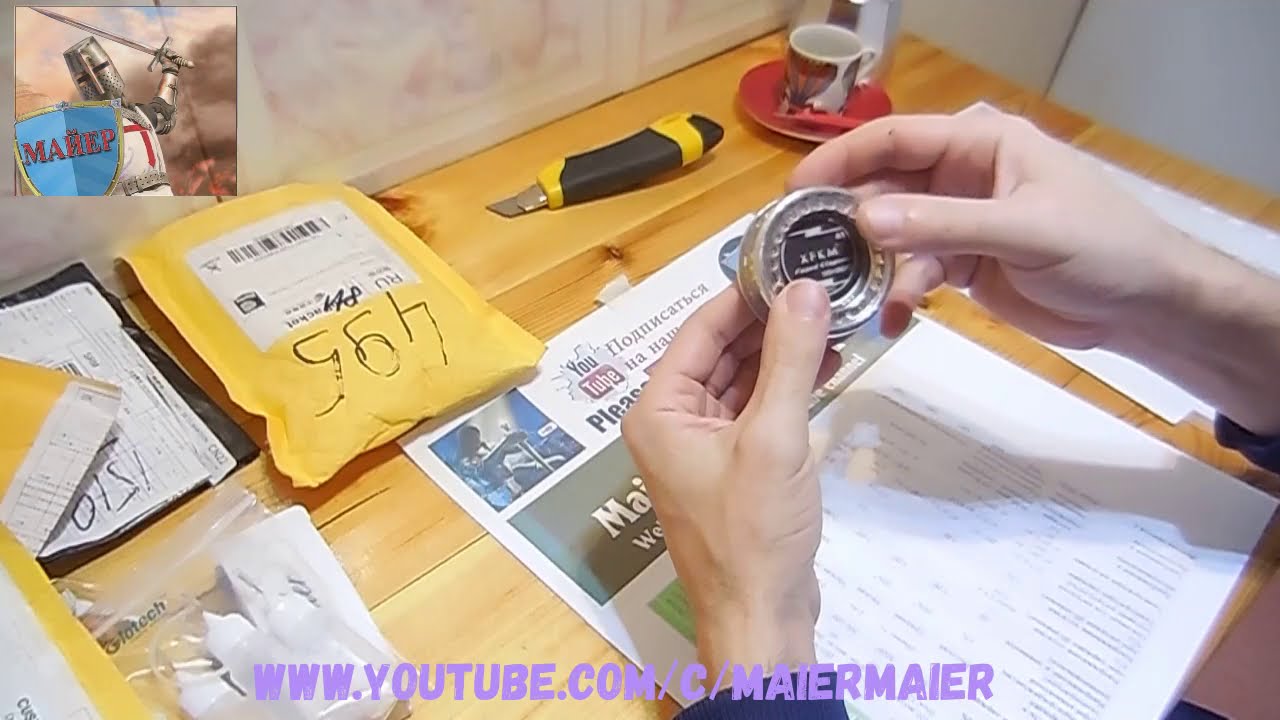This image showcases a well-organized workspace with various items strategically placed on a wooden desk, emphasizing a YouTube channel with the URL "www.youtube.com/C/MATERMAIER." A person, identifiable as a white man with a long-sleeved blue shirt, holds a small, round silver device with a black label, resembling a watch face or a metallic tin. Spread across the polished blonde wood desk are several objects: a white paper with blue and green squares and multilingual text, a yellow bubble mailer with a handwritten number "495" on it, black utility knife with yellow accents, and several other mailing and packaging supplies, including ziploc bags. To the right, a small teacup sits on a red saucer. In the upper left corner, an illustration featuring a knight with a sword beside a blue shield and the phrase "My Hip" is visible.